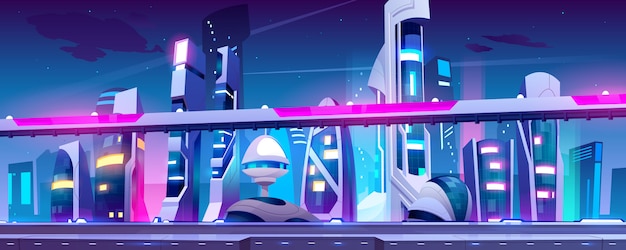This image is a detailed, animated-style drawing, depicting a futuristic nighttime cityscape. Dominated by varying shades of blue, the night sky and dark cloud formations create a mysterious atmosphere. The foreground features an elevated railway or roadway, emanating light blue, gray, and reddish-purple hues. Below this, another road crosses the image's very bottom.

In the background, an array of futuristic buildings rises against the sky. These structures exhibit unique and seemingly impossible shapes, some cylindrical and towering like open books with visible windows and lights. One notable building resembles a space capsule, adding to the otherworldly feel. The buildings are detailed with glowing purple highlights, white and yellow illuminated rooms, contributing to the impression of a vibrant, technologically advanced environment. The architecture, open and somewhat transparent, suggests a design where interiors are visible from the outside, much like a video game graphic. The overall scene is both intricate and imaginative, capturing the essence of a futuristic, cartoonish metropolis.